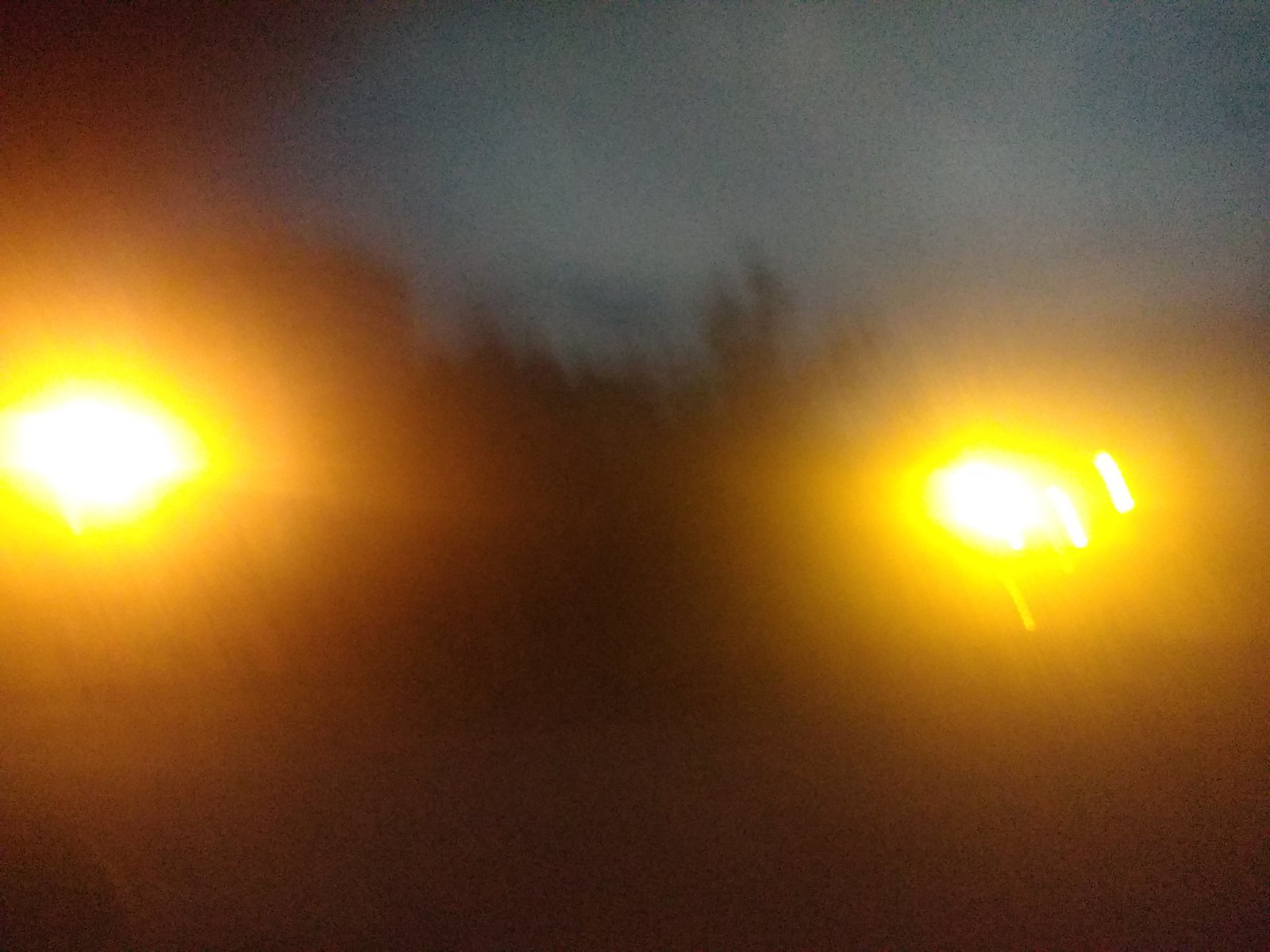This image depicts a very blurry outdoor scene, possibly taken at dawn or twilight, with a sky background that appears bluish-gray surrounded by whitish clouds. Dominating the photo are two intensely bright lights situated separately on the left and right sides. Each light features a radiant white center, encircled by progressively diminishing halos of yellow and orange hues. Interspersed within the image, starting from the midpoint and extending outwards, are multiple orange circles that seem to emanate from these lights. Silhouetted against the sky are faint outlines of trees or plants reaching upward. The lower portion of the photograph is characterized by a deep wine-red color with no discernible details apart from the vivid lights.